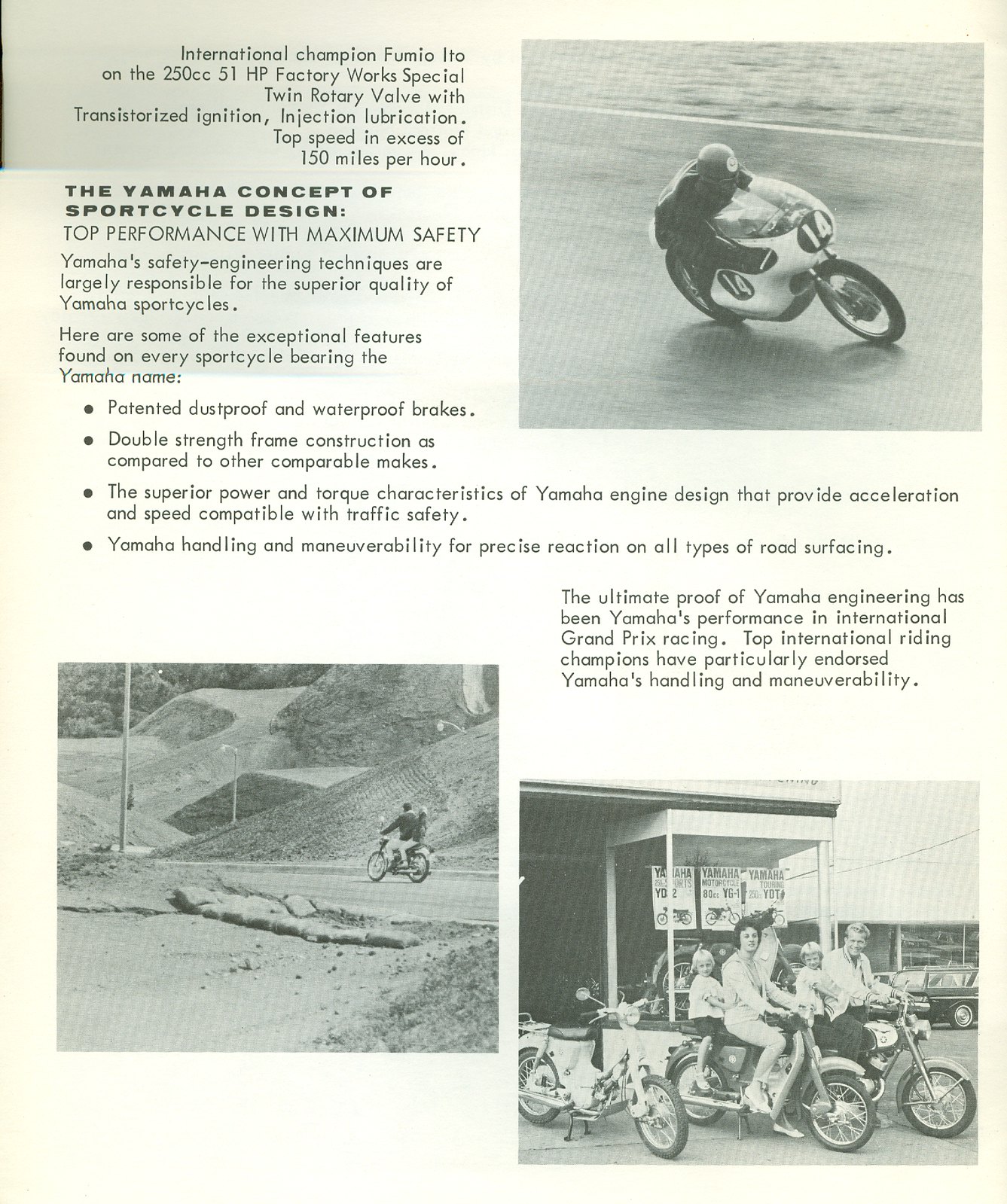This black and white image, seemingly from a vintage publication, showcases various motorcycles and their riders, emphasizing a detailed overview of a Yamaha sport cycle. At the top, there's a dynamic photograph of International Champion Fumio Ito riding a Yamaha 250cc 51HP Factory Works Special Twin Rotary Valve motorcycle. The text highlights its advanced features, such as transistorized ignition and injection lubrication, boasting a top speed exceeding 150 miles per hour. The Yamaha cycle is praised for its top performance and maximum safety, credited to Yamaha's safety engineering techniques.

Below, several photos illustrate different scenes involving motorcycles: one depicts a rider maneuvering a curve at high speed with the number 14 on the front; another shows a motorcycle on a dirt road; and the next image features a family scene with a couple riding a motorcycle alongside two children. The bottom right picture presents several motorcycles parked in front of a building, with various riders—including adults and children—posing and smiling.

The central text further elaborates on Yamaha's engineering excellence, touting features such as patented dustproof and waterproof brakes, double-strength frame construction, superior power and torque of the Yamaha engine for reliable acceleration and traffic safety, and exceptional handling and maneuverability on diverse road surfaces. These elements collectively underscore Yamaha's distinguished performance in international grand prix racing, endorsed by top international riding champions.